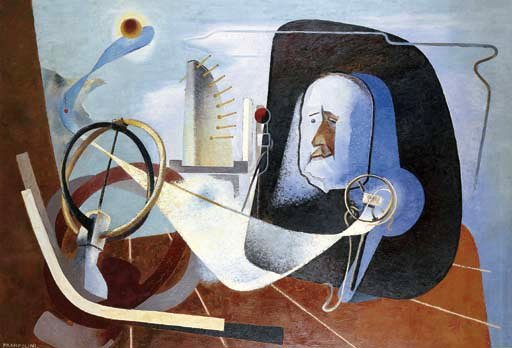This abstract painting prominently features a human figure resembling a face, slightly off-center to the right. The face, which appears to be sculpted from a black stone with white features, suggests a profile view. You can discern the eyes, nose, and mouth, evoking a sense of melancholy. The style of the painting includes an arrangement of disorganized, unsymmetrical lines, and shapes that contribute to a sense of confusion and messiness. Strong colors are used throughout, including shades of blue, black, brown, and accents of dark orange, gold, red, yellow, and white.

To the left of the face, there is a quarter-circle object with protruding elements, adding to the chaotic feel. There are also circular objects scattered within the composition; one is positioned near where the figure’s hand would be, though it's not distinctly visible due to the abstraction. Another similar circular object is placed further to the left, continuing the motif of circular shapes.

The background is a blend of blue and dark orange hues, enhancing the complexity of the image. Overall, the painting captures an abstract, possibly scientific or mathematical essence, but remains open to interpretation, embodying a blend of organized chaos and intricate detailing.